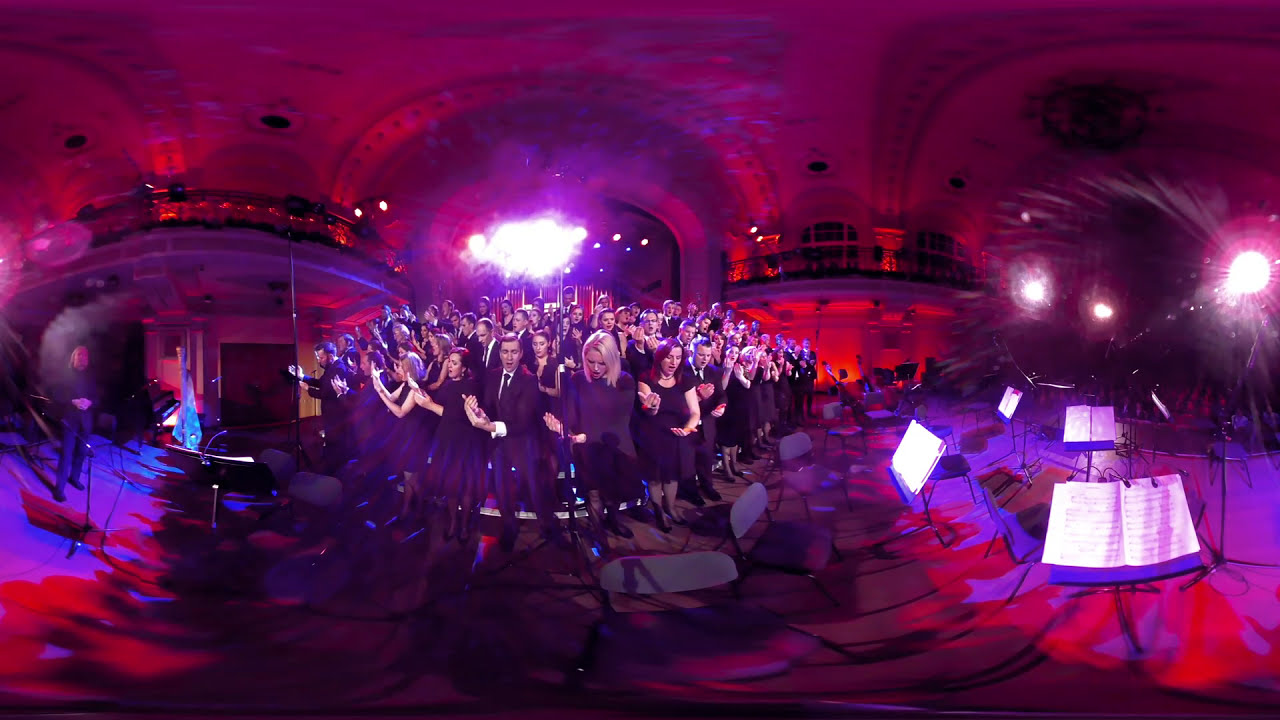The image depicts a choir of approximately 30 to 40 people performing on stage in an elaborate, large auditorium. The choir members, predominantly Caucasian, are dressed formally with men in suits and ties and women in black dresses. They are positioned on a tiered platform, getting taller towards the back, and are facing the camera as they sing. There are microphones and music stands with sheet music visible at the front of the stage. The ornate auditorium features large archways, balconies, and extensive lighting, enhancing the visual impact. Color elements such as red and purple are prominent, and a 360 imaging effect causes the colors and lights to appear to swirl, adding to the dynamic atmosphere of the performance. The audience is not visible in the image.